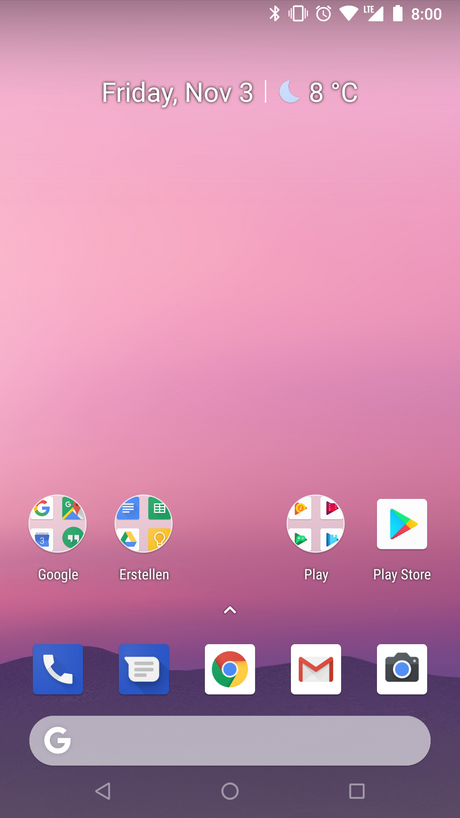Here is a cleaned-up and detailed caption for the screenshot:

---

The screenshot showcases a cell phone's home screen with a gradient background transitioning from dark blue at the top, through pink and lighter purple shades, to dark purple at the bottom two inches. The dark purple area has a jagged, mountain-like outline at the top. 

In the upper right corner, white text displays the time as "8:00." Adjacent icons indicate a full battery, strong LG signal, full Wi-Fi connectivity, an active alarm, sound status, and connected Bluetooth.

Below these icons, in the center, are the words "Friday, Nov 3" in black text. Directly beneath this, a small line separates the weather information, which features a blue half-moon icon and indicates "8°C."

The middle portion of the screen is largely blank, aside from two circular icons containing sets of four app shortcuts each. The first circle is labelled "Google" in white text. The second circle, to the right, has a similar four-app arrangement and is labelled "Play." Further to the right is the Play Store icon with the label "Play Store."

At the bottom left edge of the purple area are five icons: a blue phone, blue message, white Chrome browser, white Google Mail, and white camera. Additionally, there is a gray search bar with a small white "G" in the corner.

Finally, at the very bottom of the screen are the navigation buttons: a triangle for back on the left, a circle for home in the center, and a square for recent apps on the right.

---